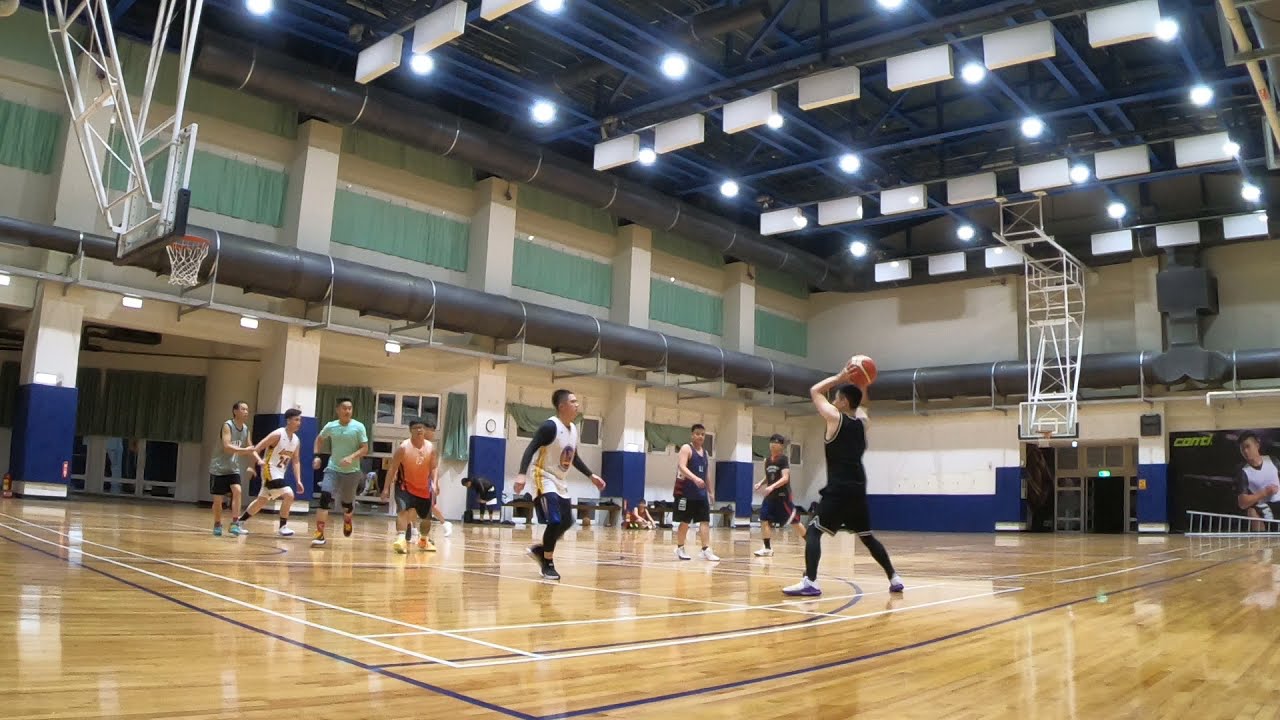The image depicts a lively pick-up basketball game taking place in a high-end gymnasium with a polished, light-to-medium brown hardwood floor. The court is marked with white and blue lines, creating a distinctive outline for the playing area. In the gym’s background, two basketball hoops are visible—one in the left upper corner and the other on the right side. The gym has tall ceilings adorned with multiple spotlights, providing ample illumination for the players. 

Centered in the image is a young man in a black sleeveless shirt and shorts, holding the basketball above his head as if preparing to pass it. Approaching him is another player in a white jersey with blue shorts, apparently ready to block the pass. Several other players with varying colored shirts—dark blue, orange, and green—are seen in the periphery, indicating a casual, non-organized game setting. One player is noteworthy for wearing a white jersey with a number on it. 

The surroundings include blue lower walls transitioning to white in the middle and upper sections, with large tubular ductwork wrapping around the gym's perimeter. An exit and entrance are visible on both the left-hand side and under the far basket. Additionally, a poster featuring an athlete can be seen in the background, further emphasizing the high-end nature of the facility.